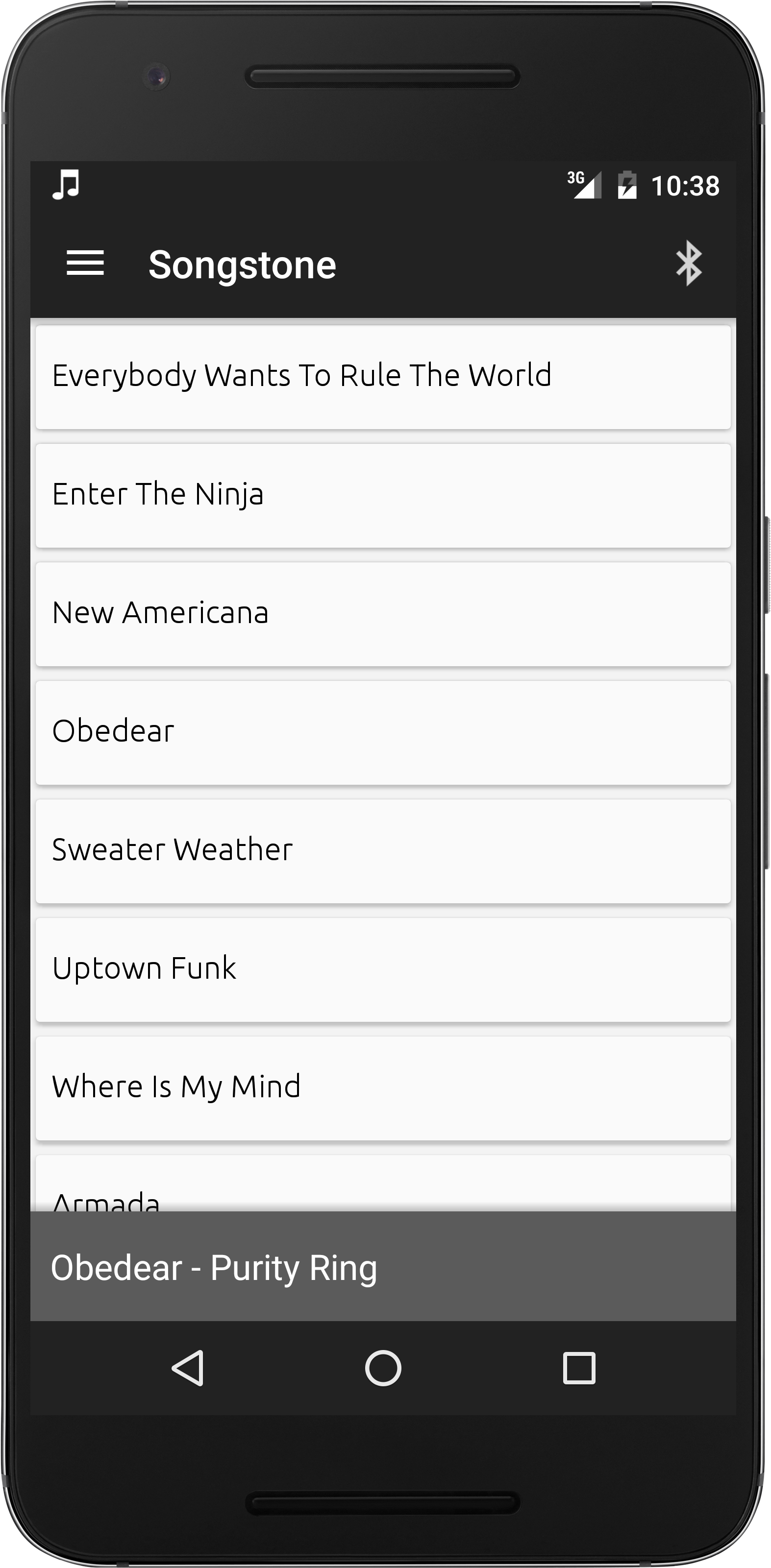The image features a smartphone screen prominently displayed in the top-left quadrant. On the screen's status bar, at the upper left corner, there is a music icon indicating that a music app is active. In the upper right corner of the status bar, the network signal icon shows connectivity to a 3G network, alongside an icon indicating that the battery is currently charging.

Below the status bar, the main portion of the screen displays a list of songs, likely from a music application or an album. The song titles visible include: "Songstone," "Everybody Wants to Rule the World," "Enter the Ninja," "New Americana," "Baby Deer," "Sweater Weather," "Uptown Funk," "Where is My Mind," and "Amada."

At the bottom of the screen, the classic Android legacy navigation buttons are visible, consisting of the back button, the home button, and the recent apps button. The overall setup suggests that the phone is in use, showcasing a selection of music tracks possibly queued for play.